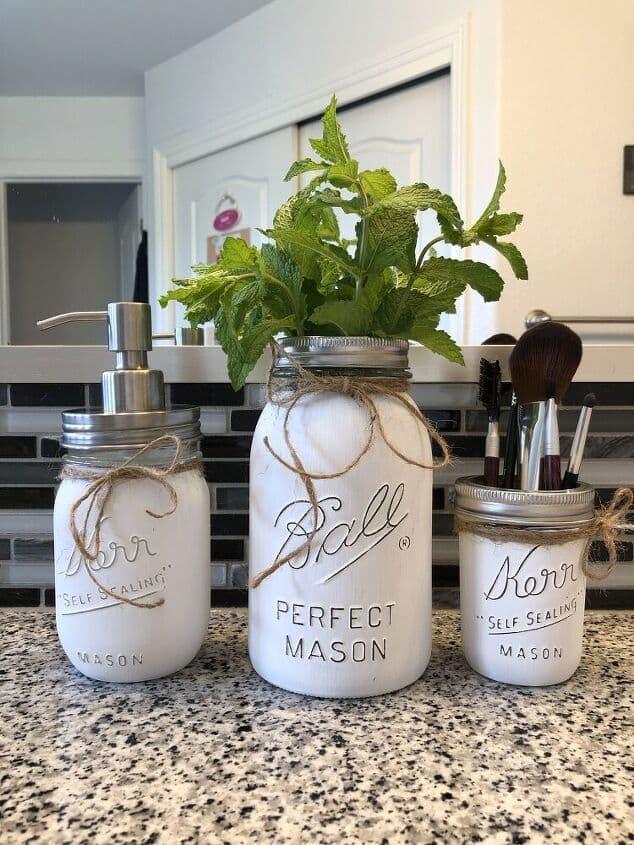This detailed photograph, captured in portrait mode, showcases a stylish countertop scene with a trio of mason jars, set against a background of black, white, and gray horizontal tiles. The surface they rest on is a granite or marble countertop, predominantly cream-colored with black and white speckles.

In the middle stands a large mason jar labeled "Ball Perfect Mason." This jar is painted white and adorned with a twine bow tied around its silver lid. It serves as a planter, housing lush green herbs—possibly mint or rosemary—with leaves that are jagged and fluffy, adding a fresh burst of greenery to the scene.

To the left is a slightly smaller jar marked "Kerr Self-Sealing Mason." Also painted white and decorated with twine, this jar has been adapted into a soap dispenser, featuring a silver pump top.

On the right, another "Kerr Self-Sealing Mason" jar, similarly painted white and garnished with twine, holds a collection of makeup brushes. The brushes are visibly inserted into the jar, supported by a silver lid with openings for the brush handles, which transition from black to dark brown bristles.

The entire setup is accented by a bright and well-lit background, featuring white walls and doors, possibly leading into another room or a closet, reflected through what might be a mirror. This chic and organized arrangement exudes an aesthetic blend of functionality and decorative charm, capturing a snapshot of domestic artistry.